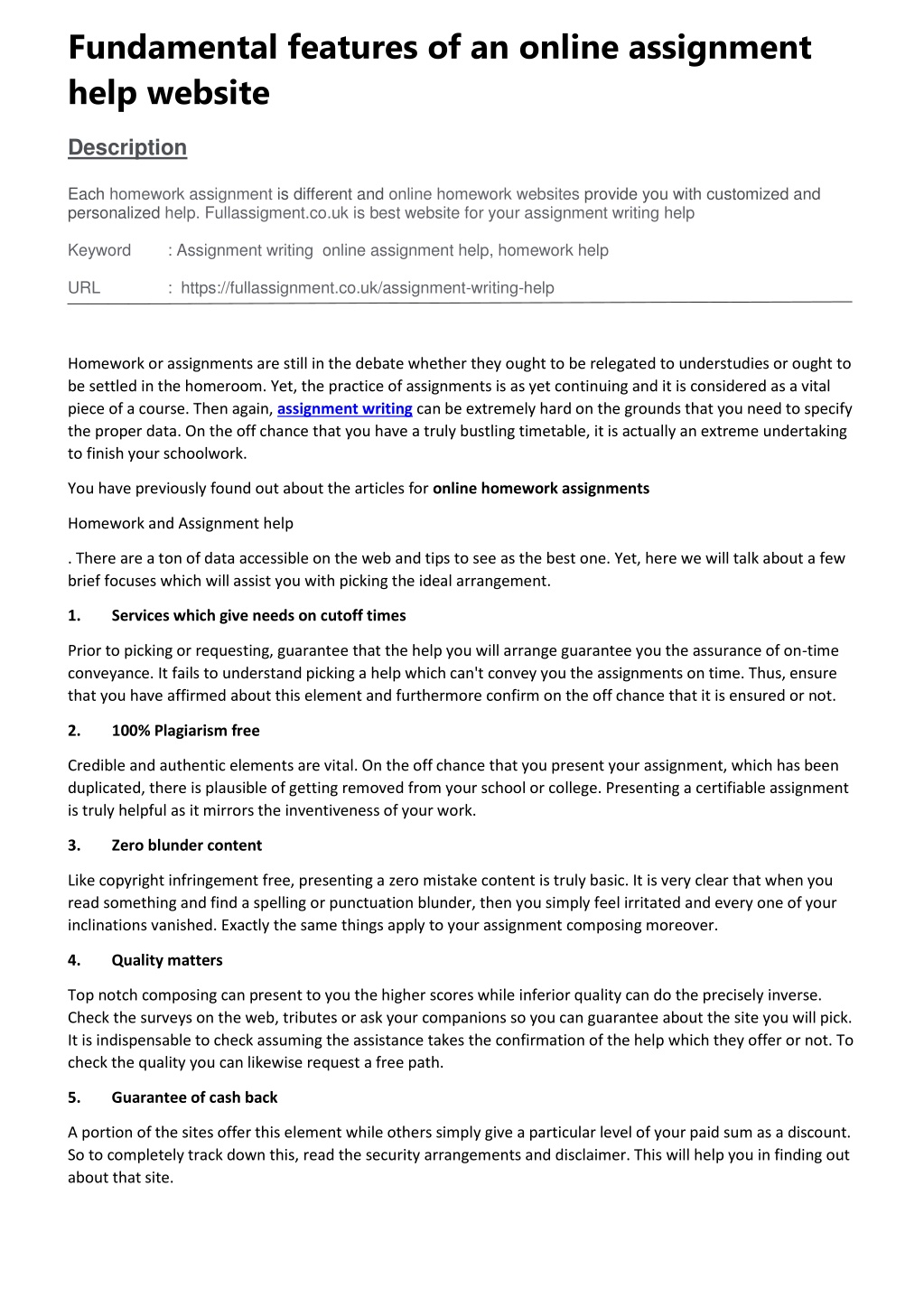Certainly! Here's a cleaned-up and detailed caption for the provided image:

---

The image displays a comprehensive webpage detailing the features of an online assignment help website. At the top, the heading "Fundamental Features of an Online Assignment Help Website" is prominently highlighted in bold letters. Directly below, a section labeled "Description" elaborates on how each homework assignment is unique and emphasizes the importance of customized and personalized assistance provided by online homework websites. It advocates for Fullassignment.co.uk as the premier platform for such assignment writing help. 

Following the description, there is a section leading with the word "Keyword," listing terms such as "Assignment Writing," "Online Assignment Help," and "Homework Help." This is succeeded by a URL segment displaying the link: "fullassignment.co.uk/assignment-writing-help." 

The webpage also includes a discussion on the ongoing debate about whether homework should be assigned to students or completed in the classroom, underscoring that assignments remain a crucial part of any course. The phrase "Assignment Writing" is hyperlinked in blue, emphasizing the challenges of conveying accurate information and managing a busy schedule to complete schoolwork.

Additional emphasis is given to "Online Homework Assignments," written in bold, as the content transitions to discuss "Homework and Assignment Help." It notes the abundance of available online information and tips to find the best help but narrows down the focus to five key categories aiding in selecting the ideal solution. These categories are identified in bold and numbered from 1 to 5, each with a corresponding description. They include:

1. Services that prioritize meeting deadlines
2. 100% plagiarism-free content
3. Zero error content
4. Importance of quality
5. Assurance of cashback

The webpage provides clear and structured information designed to guide users in choosing the most suitable assignment help service available online.